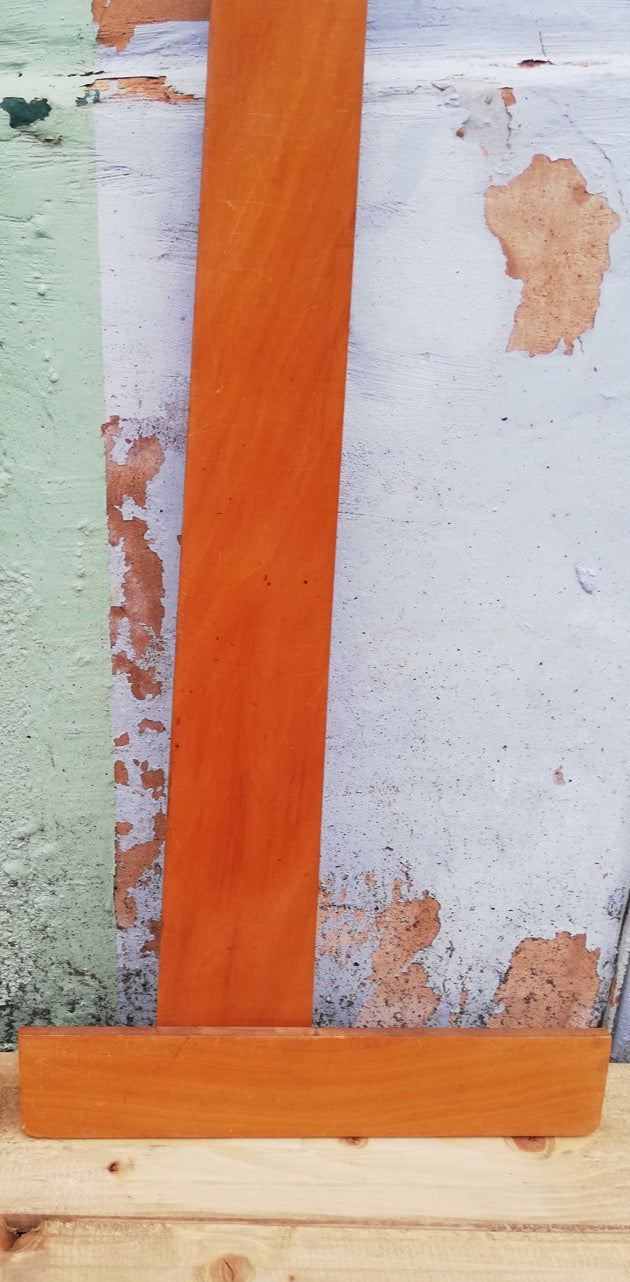The photograph depicts an outdoor construction scene during daylight, featuring a geometrically shaped tool—a large set square—propped against a deteriorating wall. The wall showcases significant signs of wear with peeling blue and white paint, revealing a salmon-colored concrete surface underneath, and apparent rain damage. Adjacent to this wall, there is a light green wall, further accentuating the contrast of the scene. The set square itself, characterized by its wood grain texture, is a striking orange-brown color and appears both vertical and horizontal, seemingly measuring the length and angle of the wall. The tool rests on a beige-colored wooden floor with visible wood grains. Additionally, the surface includes at least two layers of lighter-colored wood at the bottom and darkish brown wooden boards that seem to form a number one shape.